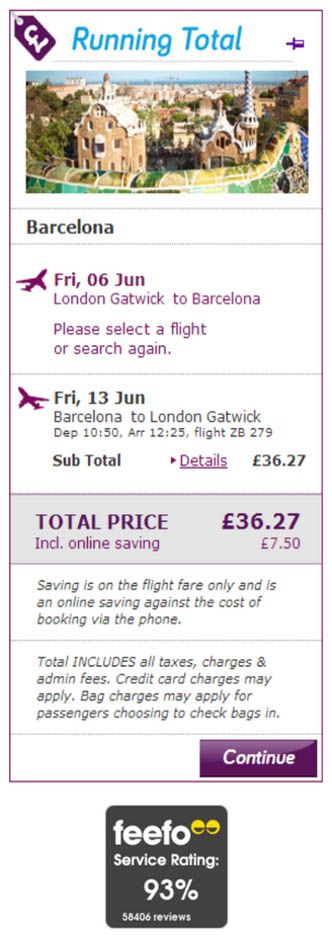This image is a detailed screenshot of a website, possibly from a travel booking site. The webpage is framed by a muted purple and brighter mauve perimeter outline. At the top, there is a tag featuring a white British pound symbol against a filled-in purple background.

Central to the image is the text "Running Total" in turquoise blue with a capital 'R' and 'T'. Below this header, the image features a graphic depiction of a cityscape, showing several large buildings with the sky and water in the background.

Further down, the text "Barcelona" is displayed prominently and in a larger, brighter font. Below this, there is a graphic of an airplane flying away, followed by the text: "Friday 06 June, London Gatwick to Barcelona. Please select a flight or search again."

Underneath, another flight detail is listed: "Friday 13 June, Barcelona to London Gatwick" in black text. Below this, it reads "Subtotal details," with "Details" in underlined purple text. The subtotal is shown as "£36.27". The section also includes a breakdown with the total price highlighted on a light gray background, "Total price including online saving," in purple text listed again as "£36.27" with an indication of savings, "You save £7.50".

At the bottom, there is white text clarifying that "Savings are on the flight fare only and is an online saving against the cost of booking via phone. Total includes all taxes, charges, and admin fees. Credit card charges may apply, and additional charges may apply for passengers choosing to check bags in."

At the very bottom of the image, a purple button with white text reads "Continue."